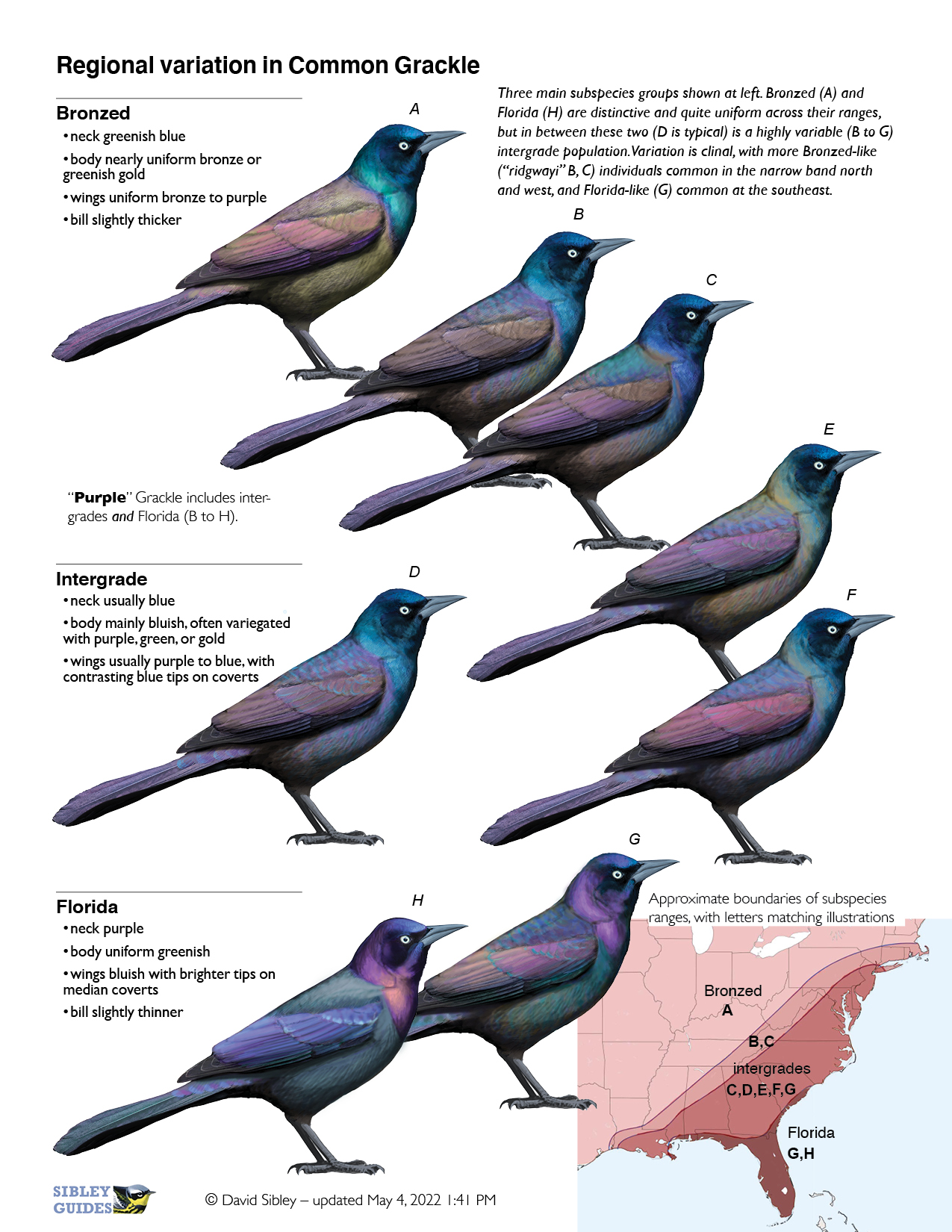The image is a detailed scientific diagram from an encyclopedia that illustrates the regional variation in the Common Grackle. It features eight labeled illustrations of the bird (A through H) arrayed in a curved shape from the upper left to lower left of the image. Each illustration highlights subtle differences among the birds, with variations in feather coloration including bronzed, purple, blue, and greenish-gold hues. The background is white, and the main title at the top reads "Regional Variation in Common Grackle" in black text. Descriptive segments on the features of three subspecies—the Bronzed Common Grackle, Intergrade Common Grackle, and the Florida Common Grackle—are found below, noting specifics such as the Florida subspecies' distinctive purple neck. An accompanying text outlines the uniform bronze to purple wings and the slightly thicker bill of the grackles. On the lower left of the image, there's a bird head logo for Sibley Guides, and on the lower right, there is a map with the legend "Approximate Boundaries of Subspecies Ranges," matching the illustrated letters to their respective geographic locations.